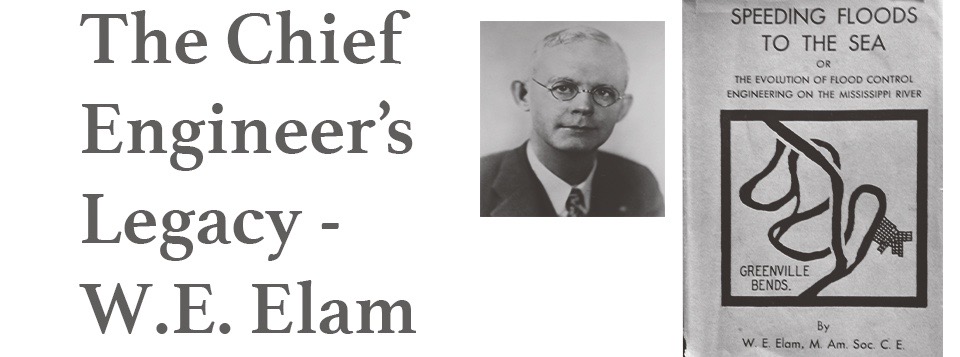The image features a monochrome collage set against a white background, combining three distinct elements. On the left, prominent gray text reads: "The Chief Engineer's Legacy" followed by "W.E. Elam." The central portion displays a black and white portrait of a middle-aged man, presumably W.E. Elam, adorned in a jacket, tie, and collared shirt, with glasses, and viewed from the upper chest upwards. To the right, there is a photograph of a book titled "Speeding Floods to the Sea or The Evolution of Flood Control Engineering on the Mississippi River," which includes a rudimentary illustration of a winding line labeled "Greenville Bends." The bottom of the book cover notes the author's credentials: "by W.E. Elam, M.M., S.O.G, C.E." The overall presentation suggests this image might be part of an article or promotional material highlighting both the author and his work on flood control engineering.